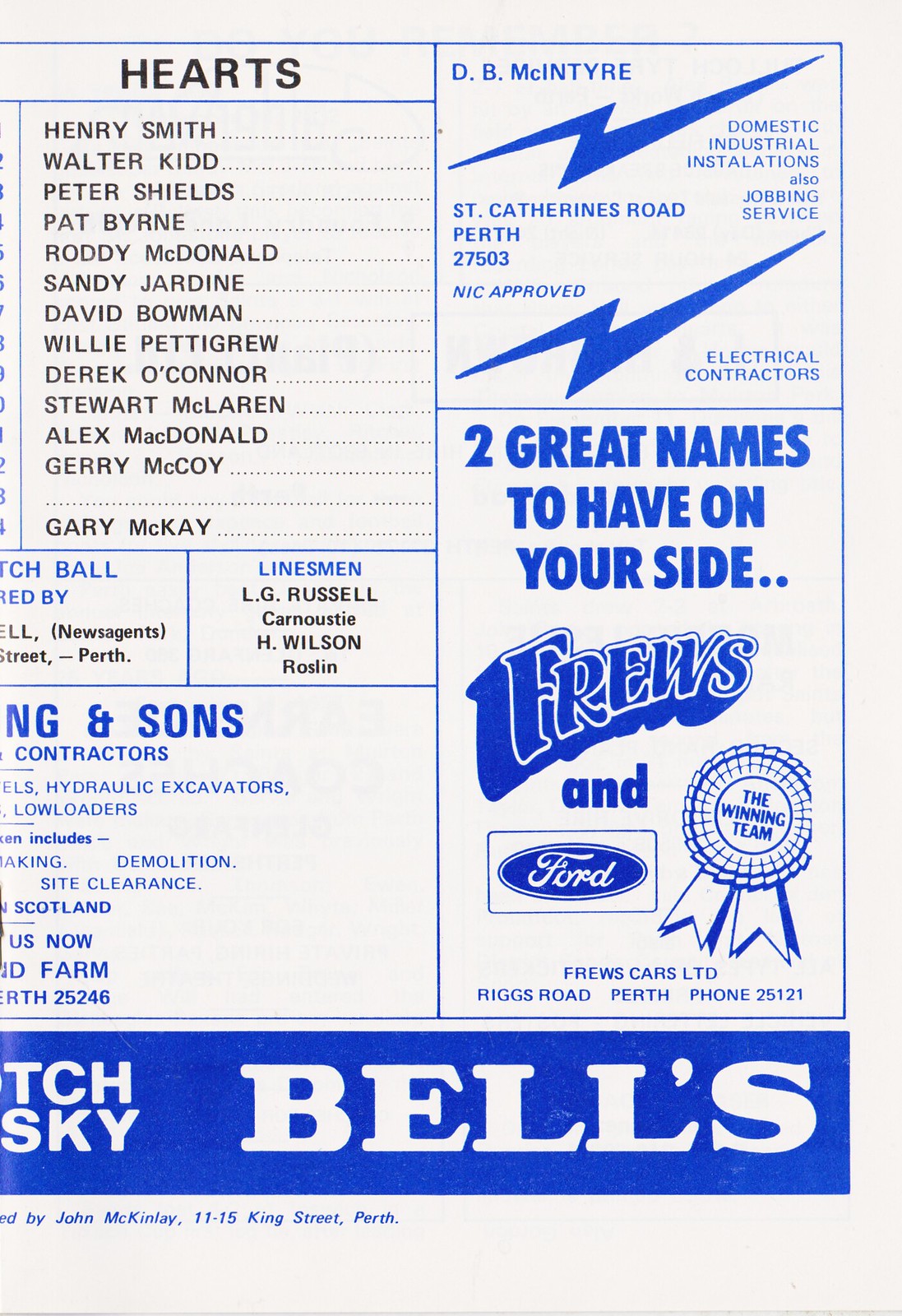This image is a portrait-oriented page from a vintage soccer club program, featuring a mix of black and blue text and graphics. On the top left, a headline in bold black text reads "HEARTS" followed by a vertical column listing the names of players: Henry Smith, Walter Kidd, Peter Shields, Pat Byrne, Roddy McDonald, Sandy Jardine, David Bowman, Willie Pettigrew, Derek O'Connor, Stuart McLaren, Alex McDonald, Jerry McCoy, and Gary McKay. Below this, several rectangles contain additional information: one partially visible section reads "News Agents" and "Perth," while another lists the linesmen as "L.G. Russell, Carnoustie" and "H. Wilson, Roslin."

Further down, an advertisement for a hydraulic excavator contractor is partly cut off, displaying terms like "Hydraulic Excavators," "Low Loaders," "Demolition Site," and "Clarence Scotland."

The top right features a blue outlined advertisement for electrical contractors, "D.B. McIntyre," including two lightning bolt graphics and text reading "Domestic Industrial Installations," "Jobbing Service," "St. Catharines Road, Perth 27503," and "NIC approved." Directly below, another ad states, "Two great names to have on your side: Fruze and Ford," featuring the Fruze Car LTD logo and an award ribbon graphic labeled "The Winning Team." Contact information reads, "Riggs Road, Perth, phone 25121."

At the bottom of the page, a blue footer bar contains the words "BELLS" in white and some other partially cut-off text. Directly beneath this footer, small blue text credits the page to "by John McKinley, 11 to 15 King Street, Perth."